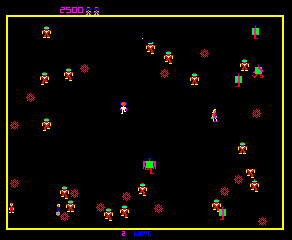This image is a detailed screenshot of an old video game, possibly from the Atari era. The game's playing field is encased within a yellow square border against a black background. In the upper left corner of the yellow square, the score is prominently displayed as "2500" in pink digital numbers with two small character icons next to it, indicating two lives left. These character icons have brown heads, blue shirts, and white bottoms. The entire screen is sprinkled with various tiny graphics: 

- Small red snowflake-like symbols scattered throughout the black background.
- Tiny characters dressed in red suits marked with a yellow 'Y,' wearing yellow shoes and green goggles.
- An array of tiny images including what appears to be a mailbox-like object with a purple bar and a green square background.
- A small spaceman character in a red suit with a green mask or shield.

At the bottom of the screen, the number "2" is displayed in pink digital numbers, with some small, blurry black or blue text next to it, which is difficult to read. The scene includes additional elements like characters in white with orange heads and some larger robots with square bodies and purple arms. Lastly, there are numerous red electronic-looking visual elements resembling flowers or sunbursts dotted across the screen.